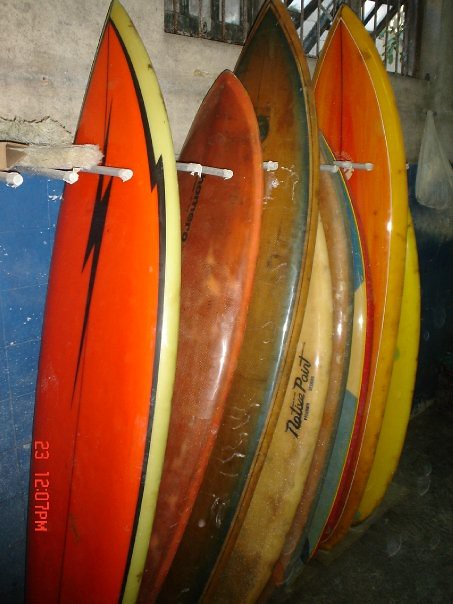This indoor color photograph showcases a vertical collection of six to seven well-used surfboards stored against a blue and slate-colored wall. Predominantly orange, with variations in burnt orange, brown, and light tan, these surfboards are held upright by white horizontal pegs protruding from the white cement or stone wall behind them. The surfboards' worn and cracked finishes reflect both their age and use. One central surfboard features the script "Native Point," though the text is somewhat hard to read. Other visual elements include a horizontal, three-sectioned window in the upper-right corner, through which daylight and the silhouettes of tropical plant branches are visible, reminiscent of modern Balinese construction. The photo, taken with a flash, captures its timestamp—23 1207 p.m.—in vertical orange digital lettering on the lower-left overlay. The dark, shadowed areas in the lower foreground add depth to the image, as well as allowing the reflective flash to highlight the surfboards' surfaces.